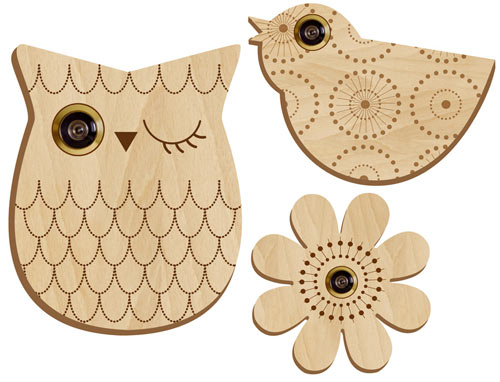The image depicts three intricately crafted thin wooden pieces of art set against a white background. Each piece features a common element of a fish-eye viewer or button as part of its design. Starting from the bottom right, the first piece is a flower with eight circular petals arranged around a black button in the center. Concentric circles with dots extend from the button, mimicking the inner petals of a real flower. Above the flower, there is a bird, which appears to be nesting. The bird’s eye is a similar fish-eye viewer surrounded by concentric circular decorations that give an illusion of a Ferris wheel. Lastly, on the left, there is an owl carved in a shape somewhat reminiscent of a pineapple. It has a closed painted eye and an open eye made from a fish-eye viewer encircled by a green ring. The owl's feathers are detailed with brown dots, and half-circle shapes at the top represent its hair. Each piece remains in its natural light wood color, amplifying the intricate designs and thoughtful use of buttons and viewers to create unique focal points in the artwork.